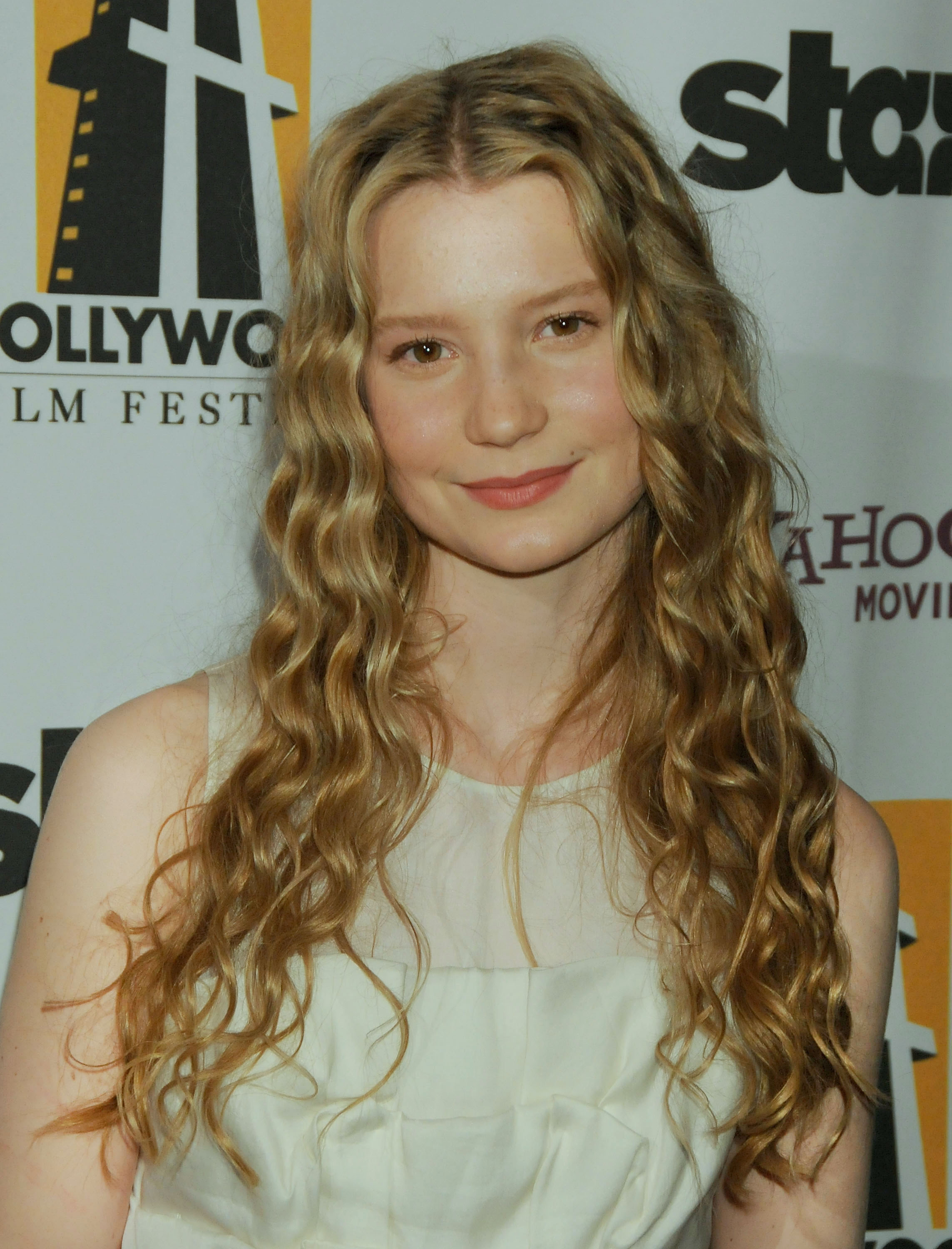In this photo, we see a young woman, likely in her early 20s, with long, wavy blonde hair cascading down to her chest. Her hair, parted in the middle, features light brownish blonde hues that match her dark eyes. She is wearing a sleeveless white top and stands in front of a promotional backdrop indicative of a red carpet event, such as the Hollywood Film Festival. The backdrop is predominantly white and adorned with various logos and text in black, orange, and purple. Key elements on the banner include a large letter "H" and a movie reel against an orange background, the words "Hollywood Film Fest," and "Yahoo! Movies." The logos and text are repeated in several places, providing a busy and dynamic background that emphasizes her presence at an important industry event.